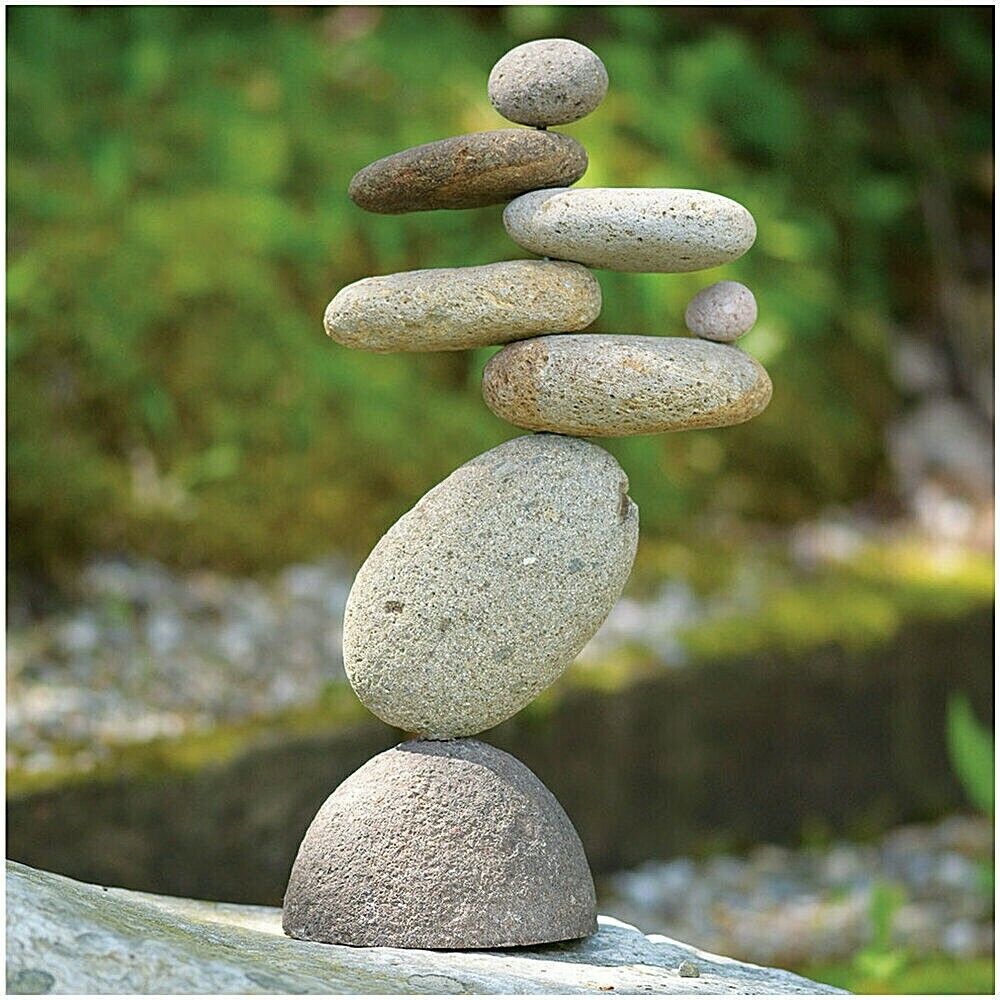In this photorealistic image of a meticulously crafted rock sculpture, eight smooth stones of varying sizes are artistically stacked on top of a flat-bottomed, domed stone base, creating an almost impossible yet beautifully balanced structure. Closer inspection reveals a metal rod and glue, ensuring the stability of this stacked formation, showcasing the intricate artistry behind it. The stones range in color from light gray to brown, with one dark brown stone positioned second from the top. The stack is set on a large, slightly green-tinged white boulder, which stands at the bottom foreground of the image. The background, though slightly out of focus, reveals a serene natural setting with a small stream running through the center, flanked by a rocky shore on either side, and lush green trees and shrubbery providing a tranquil backdrop.